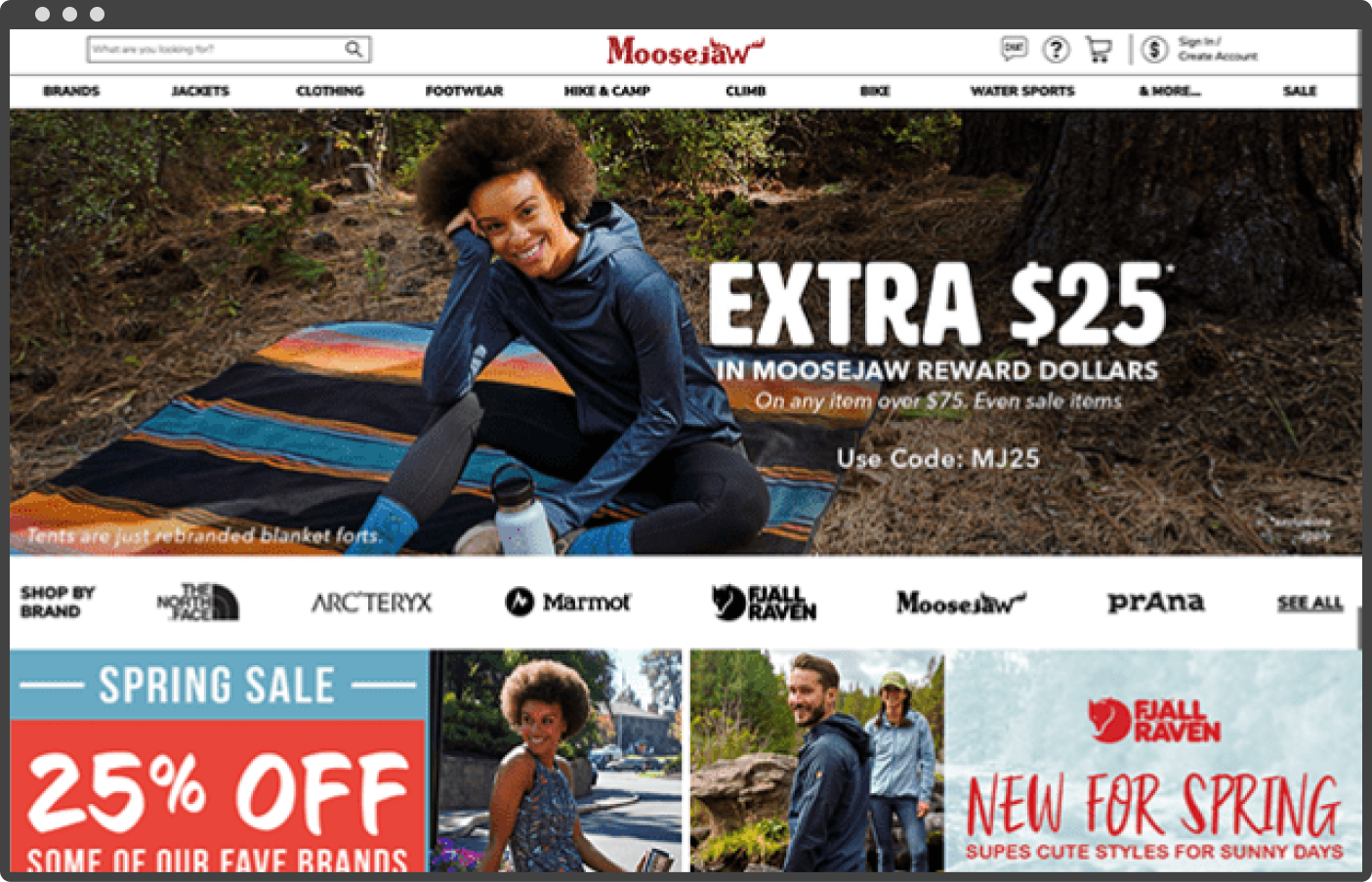The image showcases a web page from Moose Jaw. At the top center, the page title "Moose Jaw" is prominently displayed in bold red ink. 

Below the title, there's a photograph of a woman of color with curly brown hair. She is seated on a black, blue, and orange striped blanket in a wilderness setting. She is wearing a dark blue hooded shirt, black leggings, and blue socks, with a white water bottle positioned in front of her. 

Adjacent to the image, large white capital letters advertise an "EXTRA $25." Directly underneath, the text states, “in Moose Jaw reward dollars on any item over $75, even sale items. Use code MJ25.”

Further down the page, there is a section titled "Shop by Brand," featuring clickable logos and names of popular outdoor brands such as The North Face, Arc'teryx, Marmot, Fjällräven, Moose Jaw, Prana, and an option to "See All."

The section is followed by four individual image blocks. The first block announces a "Spring Sale 25% Off." The second block shows the same woman from the earlier image, but this time she is wearing a different shirt and is pictured in an urban street scene. The third block features a man and a woman together in a wilderness setting, and the final block invites users to explore "New for Spring" items.